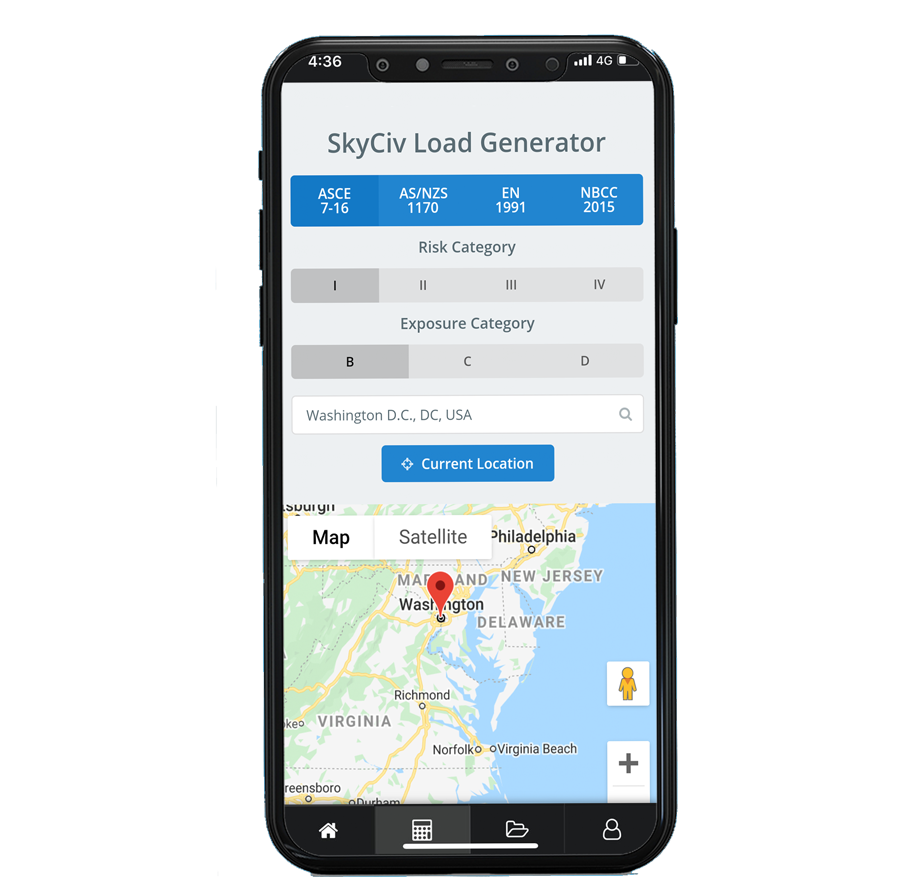Detailed Caption: 

The image showcases a screen from the SkySIV CIV Load Generator software, with version 436. The software supports various structural standards including ASCE 7-16 and AS/NZS 1170. The ASCE standard is prominently highlighted in blue, featuring different shades where "E" is dark blue and the rest of the label is light blue. The interface also includes options for different load codes like EN 1991 and NVCC 2015, especially catered for a Risk Category, which is marked with "1" in gray highlight. Additionally, the Exposure Category is presented with options labeled as 234, with "B" in gray highlight, along with "C" and "D."

The top section of the interface includes a search bar, with "Washington, D.C., U.S.A." entered, accompanied by a magnifying glass icon. A blue rectangle labeled "Current Location" becomes visible, flanked by a white map that provides a satellite view. There's also a location pin icon placed near Washington, D.C. 

At the bottom of the screen, there are several utility icons: a picture of a house, a calculator highlighted in gray, a file folder, and a profile icon, indicating various functionalities within the software.